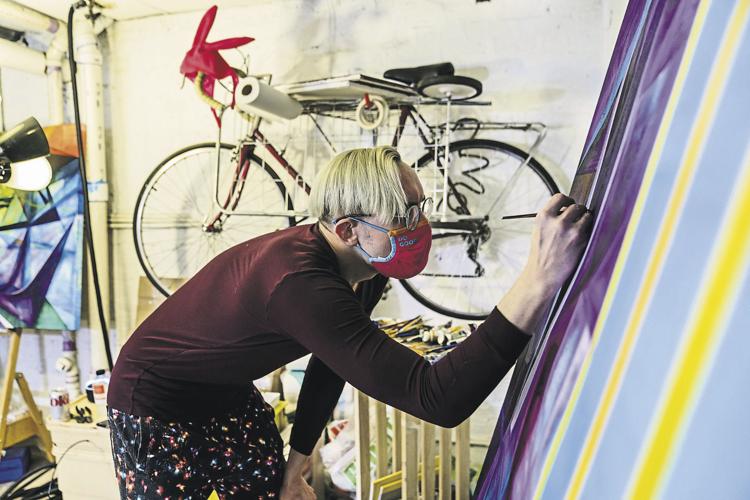The photograph captures an artist's studio with a tan wall in the background, reminiscent of a garage or storage area. Dominating the foreground, a slender man with flowing blonde hair cascading to the right side of his face is intensely engaged in his work, bent over with one hand on his knee and the other hand wielding a paintbrush or pencil. He is dressed in a long-sleeve maroon shirt and baggy black pants adorned with colorful patterns, and he wears a red face mask and round glasses, possibly to protect against fumes. The large canvas he's working on features colors of dark purple, light purple, light blue, and stripes of yellow, though the exact details of the artwork remain obscured.

The background illustrates an industrious and creative environment. A 10-speed bike with red bars and yellow-wrapped curved handlebars hangs on the wall, doubling as storage for a grocery cart, paint canvases, and a roll of paper towels. Exposed pipes and electrical cords contribute to the industrial feel. On the left, an easel supports an abstract painting, while additional easels and finished artworks are scattered around. A crate, serving as storage for paints and brushes, is also visible, adding to the organized chaos of the studio space.